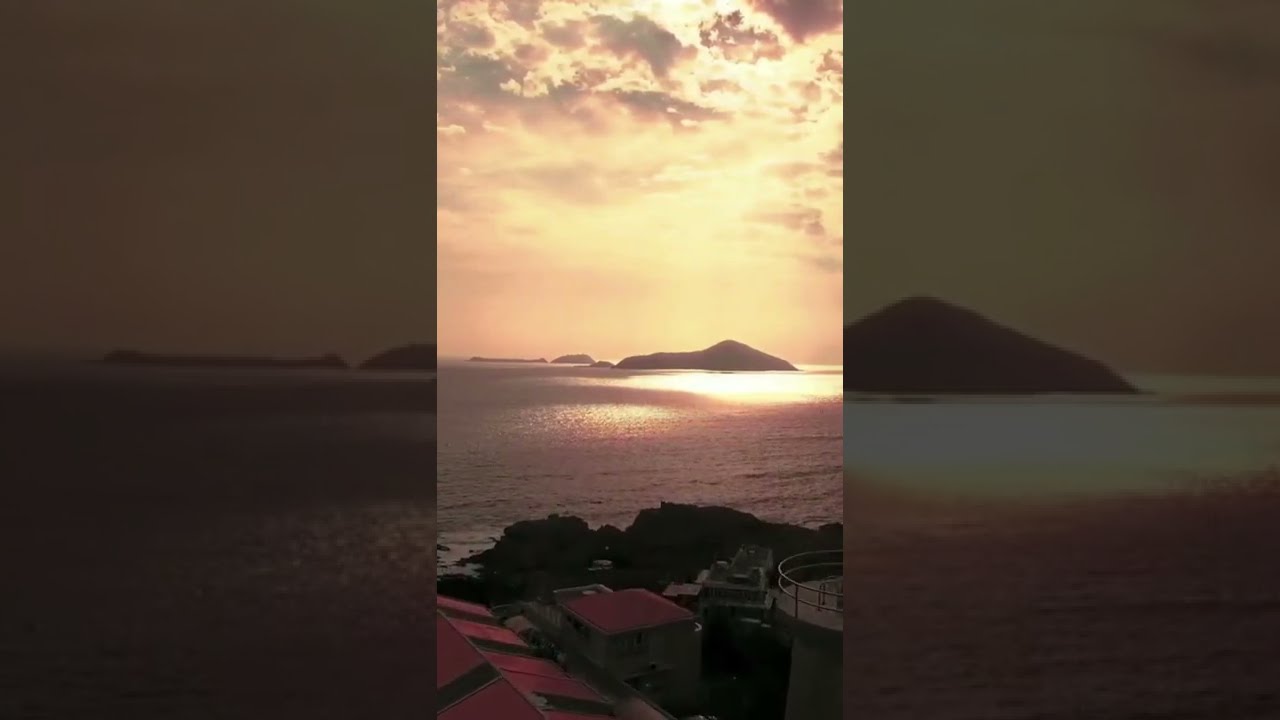This is a photograph taken during twilight, likely sunset, capturing a serene oceanic waterway with the sun's reflection shimmering on the darkened surface. The sky is strikingly dramatic, filled with fluffy, gray clouds partially obscuring the fading light, providing a golden hue. In the distant horizon, multiple hilly islands are visible, with one particularly larger and closer than the rest. The foreground shows a rocky coastline shadowed in darkness, sprinkled with large dark rocks and a few trees. Among these rocks, there's the faint outline of a cooler, suggesting someone's presence near the shoreline. Additionally, you can spot some buildings with pinkish roofs nestled along the coast, their details blurred by the shadows, enhancing the overall tranquil and moody atmosphere of this twilight landscape.